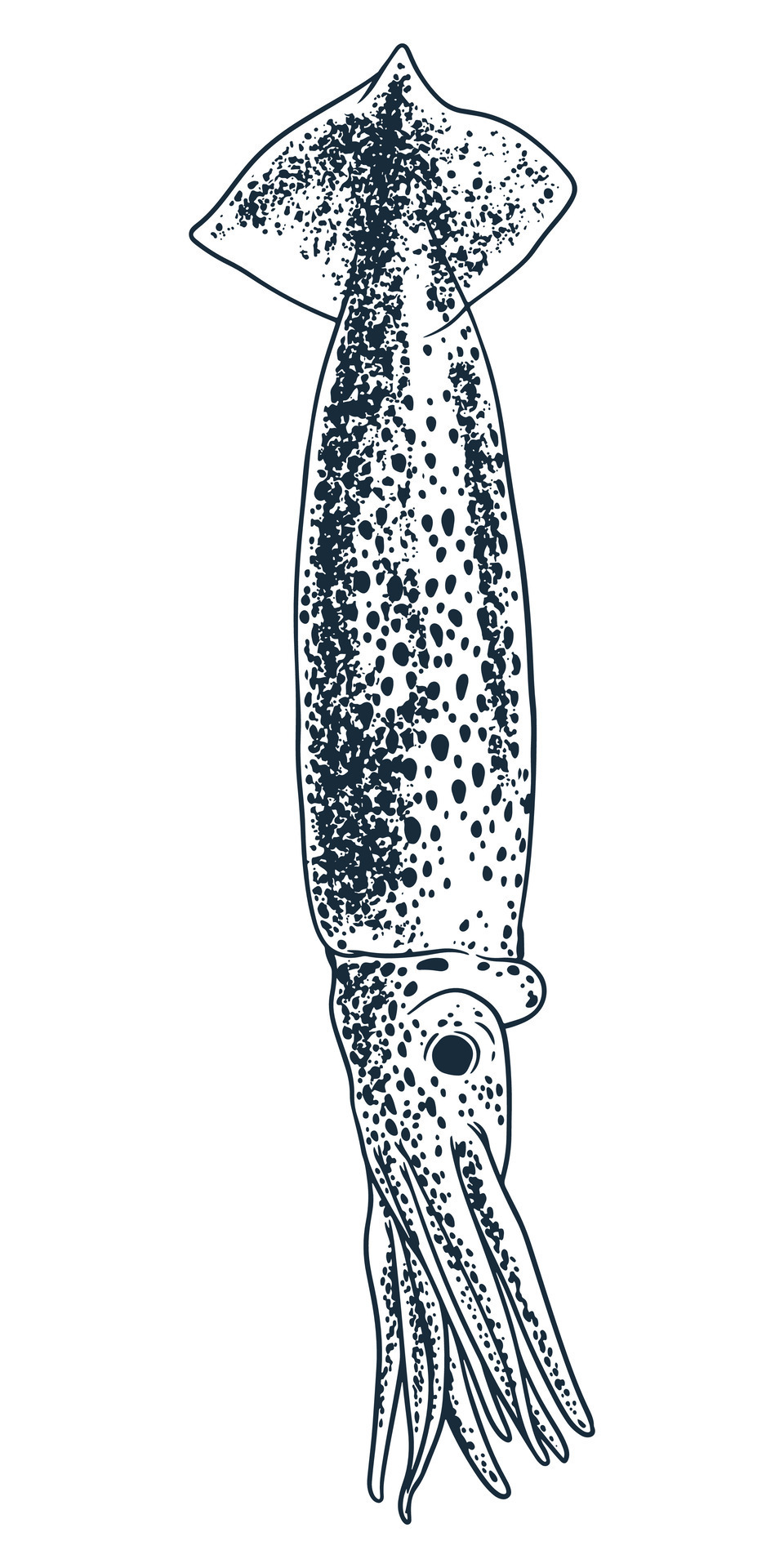This image is a detailed black-and-white drawing of a squid, created using black pencil or marker. The squid is depicted hanging upside down, with its tail at the top and its face oriented toward the bottom. The squid's cylindrical body ends in a tail that fans out into three points. One prominent eye is visible next to its many tentacles, which emerge from the front of its face. The body, face, and tentacles of the squid are all covered with black spots and blotches. The size of the drawing is approximately 12 inches (one foot) long. The background is entirely white, enhancing the contrast of the black markings. The squid appears to have a separation between its head and body, with little variation in thickness from head to body. Notably, there are spaces between spots on the fins, adding to the intricacy of the illustration.